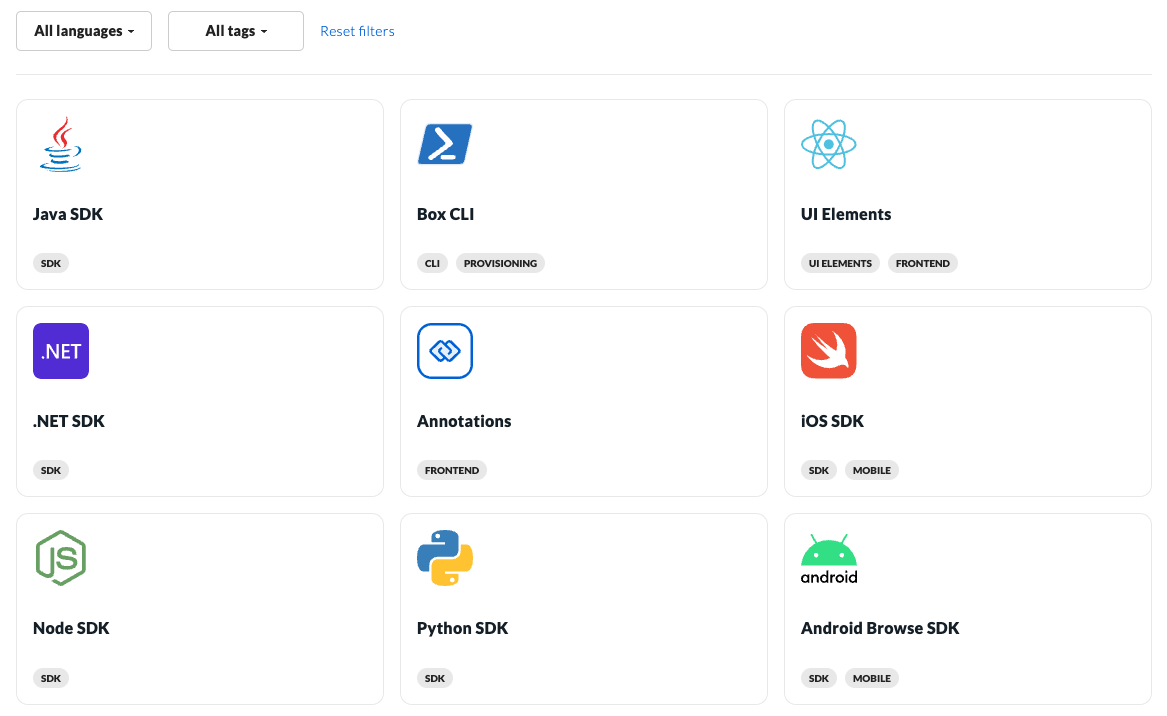The page features a clean white background. At the top left, there are two light gray-outlined rectangles - the first rectangle contains bold black text that reads "All Languages" with a downward-pointing arrow indicating a dropdown menu. The second rectangle is similar but reads "All Tags," also with a dropdown menu. To the right of these rectangles is blue text that reads "Reset Filters."

Below this header section, the content is organized into a grid of three rows, each containing three squares outlined in very faint gray. 

- In the first row, the first square displays a small blue and white cup and saucer with red steam rising from it, positioned in the upper corner. Beneath the icon, in black text, it says "Java SDK."
- The second square in this row has a blue background and a white directional arrow pointing to the right. Beneath the arrow, in black text, it reads "Box CLI," followed by "CLI Provisioning."
- The third square features a blue atom icon. Below it, in black text, it says "UI Elements" with "UI Elements Front End" listed underneath.

In the second row:
- The first square is purple with white text that reads ".NET." Beneath this, it says ".NET SDK" in black text, with "SDK" listed below that.
- The second square has a white background outlined in blue, with a blue sideways "S" icon. Beneath the icon, in black text, it reads "Annotations," followed by "Front End."
- The third square is red with a white outline of a diving bird. Underneath this, it says "iOS SDK" in black text, followed by "SDK Mobile."

In the third row:
- The first square features a green polygon with white text that reads "JS" in the upper left corner. Beneath this, it says "Node SDK" in black text, with "SDK" underneath.
- The second square displays a blue and yellow snakes icon in the upper right corner. Underneath it says "Python SDK" in black text, followed by "SDK."
- The third square features the top of a green android robot head with two antennas and dot eyes. Beneath this, in small black text, it reads "Android." Below that, it says "Android Browse SDK," followed by "SDK Mobile."